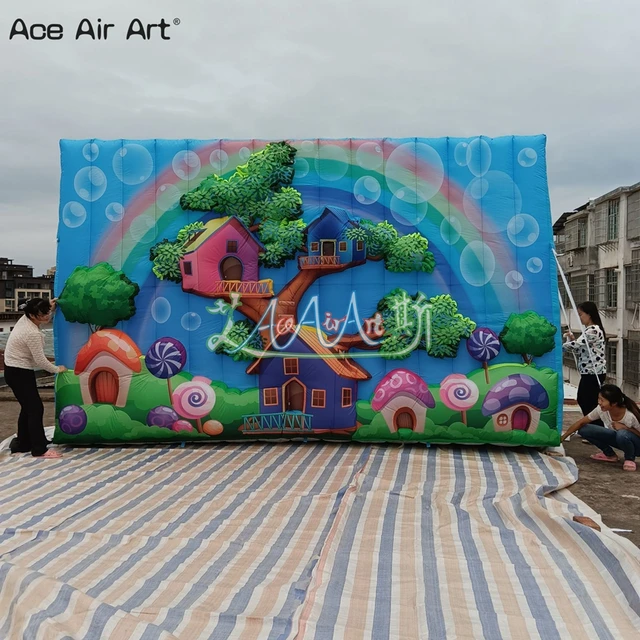In this image taken on a cloudy, overcast day, three women are setting up a large, colorful canvas backdrop outdoors. The ground in front of the backdrop is partially covered by a large, striped blanket with blue, white, and beige stripes. The canvas itself, held taut by one woman on the left and two on the right, features a vibrant, cartoon-style treehouse scene. The treehouse design is lively, with a main blue house on the ground, a pink house further up the tree, and another blue house higher still. Surrounding the treehouse are whimsical elements like bubbles, a rainbow, and various candies and lollipop-like items, giving it a Wonka-esque feel. The backdrop also includes smaller blue and pink houses resembling cornflowers and mushroom houses. In the top left corner of the canvas, the text "Ace Air Art" is written, possibly with a copyright symbol, while the entire scene is framed by old buildings on either side and set against a backdrop of overcast skies.